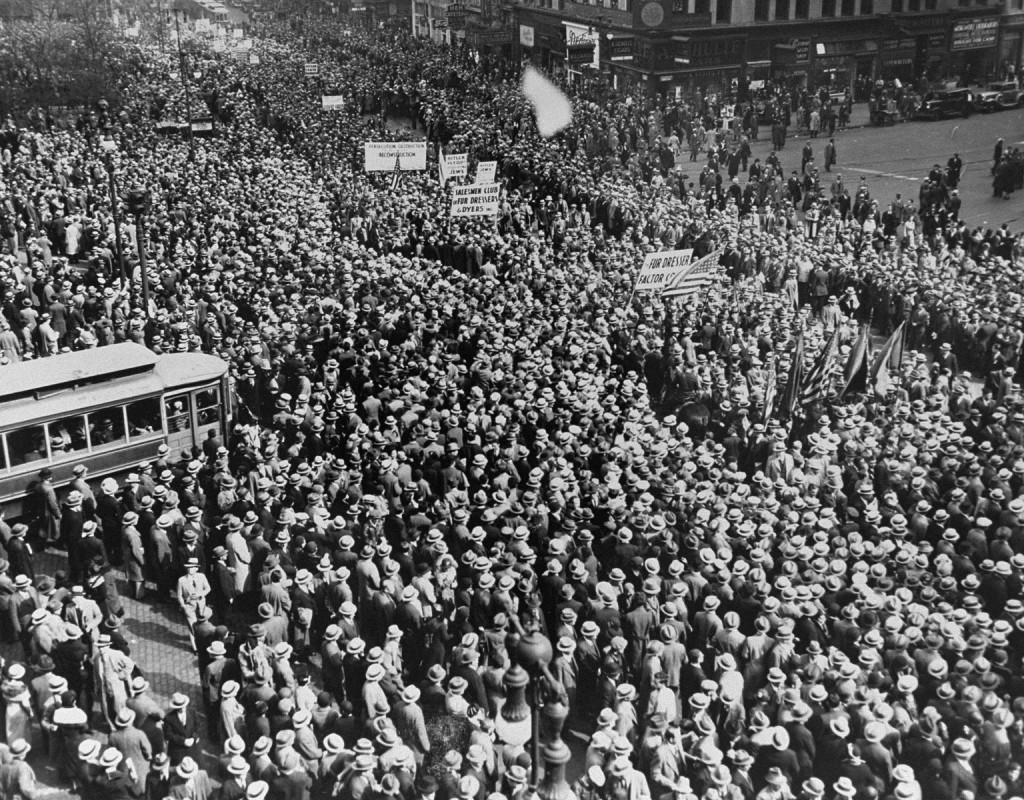This black and white photograph, likely taken in the early 1900s, captures a large political rally or protest in an American city. A mass of predominantly male attendees, clad in old-style suits and white top hats featuring a black band, fills the scene. The crowd, numbering in the hundreds or possibly thousands, appears organized into several distinct sections. American flags and various unidentifiable signs are prominently displayed, adding to the march's patriotic fervor. The backdrop features urban architecture, including visible buildings and parallel-parked cars in the top right corner. To the left, a tram stands amidst the crowd, marking the presence of public transportation at the time. The uniform attire and the historical context depicted by the hats and coats evoke a striking sense of unity and purpose among the demonstrators.